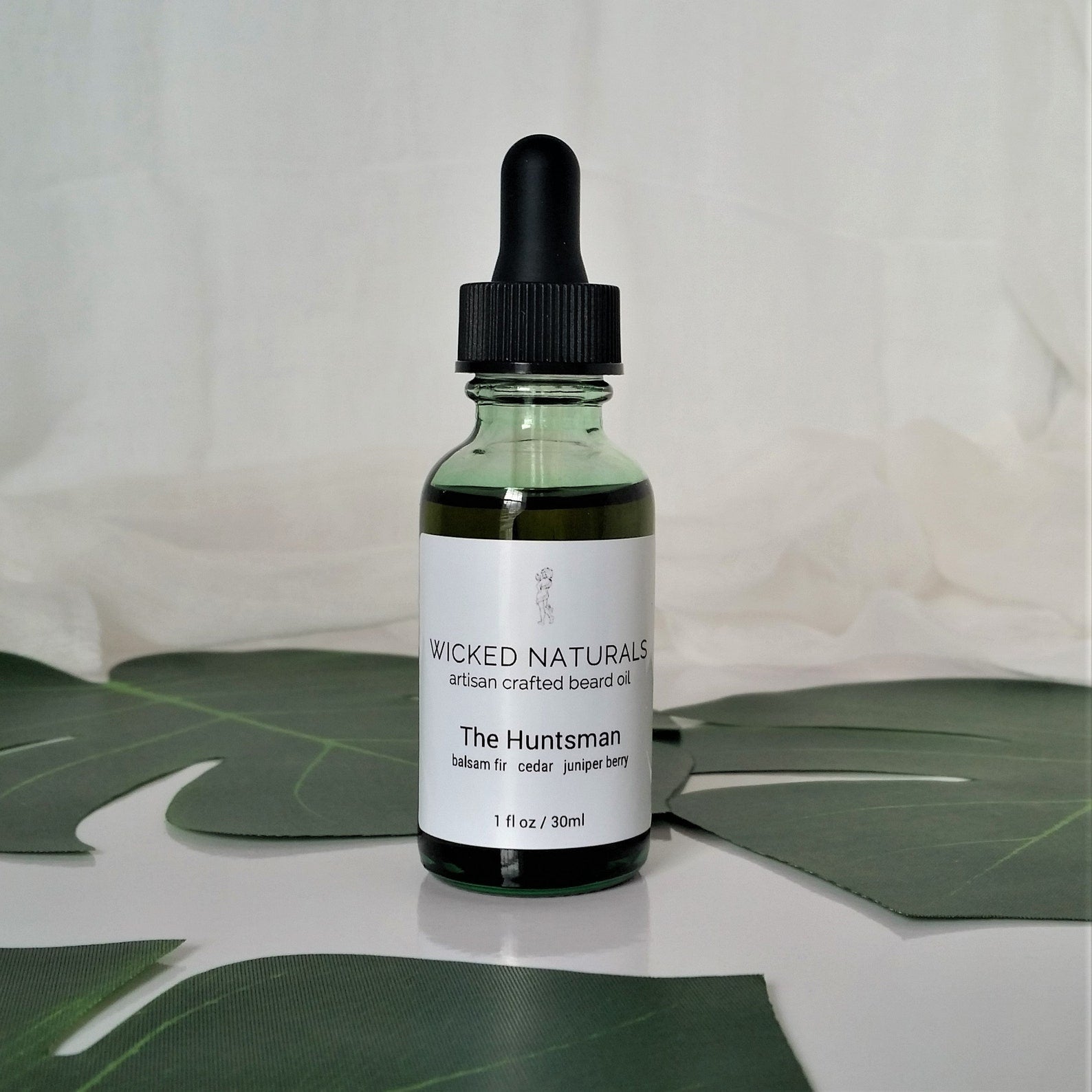The image showcases an advertisement-style presentation of a bottle of beard oil against a white background. The product, by Wicked Naturals, is called "The Huntsman" and is artisan-crafted. The clear glass dropper bottle, featuring a black cap, contains one fluid ounce (30 milliliters) of dark green beard oil, which is a blend of balsam fir, cedar, and juniper berry. The bottle is prominently labeled with a white label that reads "Wicked Naturals Artisan Crafted Beard Oil - The Huntsman." The setup includes artistic cutouts of dark green leaves, enhancing its rustic and natural aesthetic, and rests on a pale white fabric surface for a clean, minimalistic look.